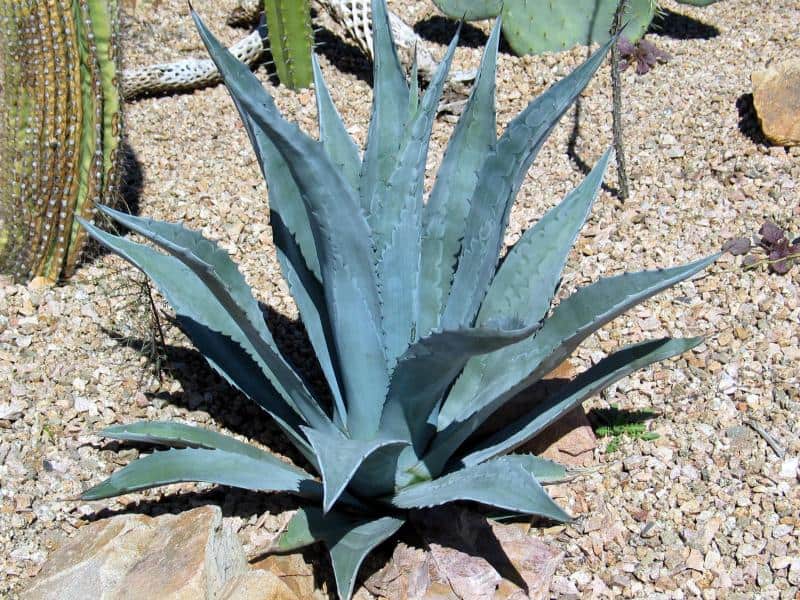The photograph is a rectangular image taken outdoors in a cactus garden on a bright, sunny day. The central focal point is a large, blue-green cactus, which may be an aloe vera, with long, pointy leaves featuring small scales or spikes along their edges. This main cactus, slightly below the center, displays a variety of leaf sizes; the shorter, thicker leaves are oriented toward the viewer, while the taller, thinner leaves extend to the sides and the back. The ground is covered entirely with small tan and brown rocks and pebbles, with some larger rocks scattered around, particularly in the bottom left of the image.

In the background, multiple types of cacti are visible: to the left, another cactus base extends out of the frame, while near the top center, a tall, elongated cactus with numerous spikes is seen. To the right of it, a rounded cactus with flat disk-like leaves is distinguishable. Additionally, there appears to be a white, snake-skin-like object near the center top of the image, though its details are indiscernible. The overall color palette of the photograph includes various shades of green, brown, and tan, enhanced by the clear sunlight that also casts subtle shadows behind the main cactus.